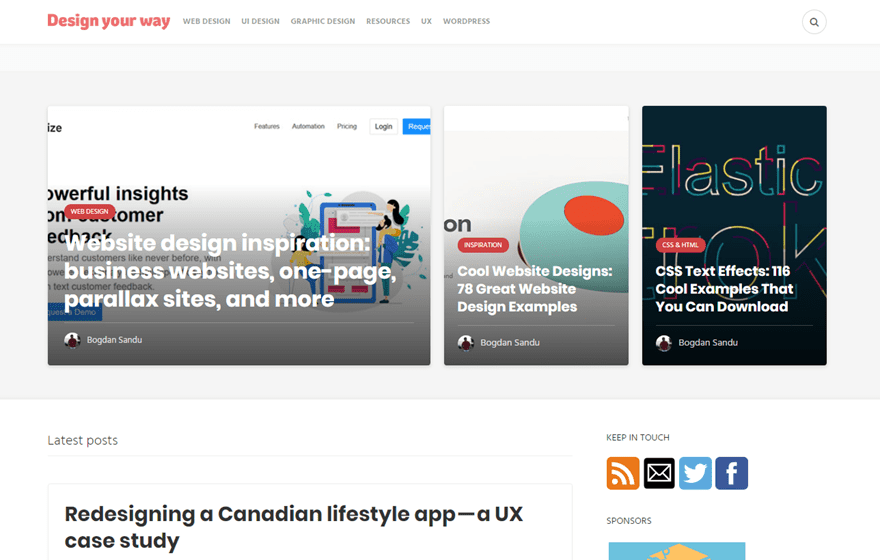The screenshot captured in the image is horizontally rectangular and appears to be from a design-focused website. In the upper left corner, set against a red background, is the website's logo or motto: "Design Your Way." To the immediate right of this text lies a navigation bar with selectable options labeled as "Web Design," "UI Design," "Graphic Design," "Resources," "UX," and "WordPress." On the far right end of this navigation bar, there's a search icon for user convenience.

Beneath the navigation bar, three images are aligned side-by-side. The left-most image is horizontally rectangular and features the text "Website Design Inspiration: Business Websites, One-Page, Parallax Sites, and More." The middle image, which is vertically rectangular, showcases the title "Cool Website Designs: 78 Great Website Design Examples." The third image, also vertically rectangular, is labeled "CSS Text Effects: 116 Cool Examples That You Can Download."

Following these images, there is a section titled "Latest Posts," under which the article "Redesigning a Canadian Lifestyle App - A UX Case Study" is listed prominently.